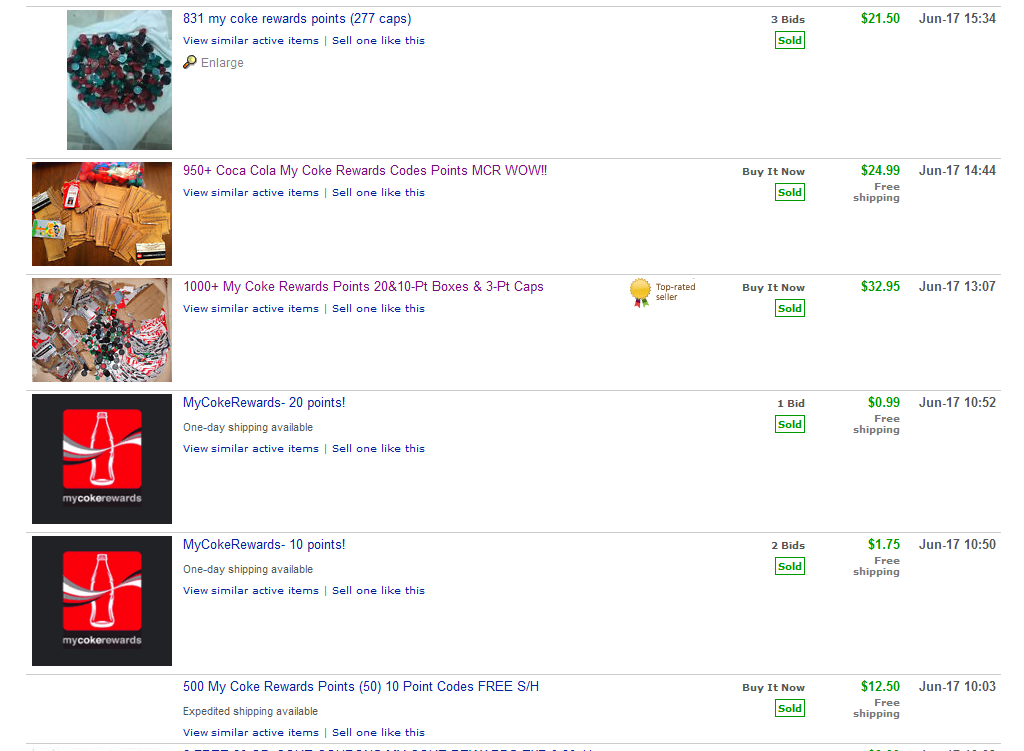This webpage showcases various listings for "My Coke Rewards" points. The layout features multiple horizontal sections, each rectangular in shape and offering different rewards items for sale. 

At the top section, there is an image depicting various Coke bottle caps, possibly placed in a container, accompanied by text that highlights "831 My Coke Reward points" along with "277 caps." To the right of the image, the listing includes the selling price marked at "$21.50" in green text. Additionally, a small green box notes that the item has been sold, and the date of sale is displayed in black text below.

The subsequent section shows another reward option, specifically "950+ Coca-Cola My Coke Reward codes points." This listing includes a "Buy it Now" option, and like the previous entry, it indicates the sold status with "Sold" in green text, a price of "$21.99" also in green, and "Free Shipping" in light gray text. The date is again noted in black beneath the details.

Scrolling down, a total of six such sections are presented, each offering varying amounts of My Coke Rewards points, caps, and codes. For example, the third section features another collection of caps and boxed codes, each priced individually. Other sections include offers like "My Coke Rewards 20 points" and "My Coke Rewards 10 points," each accompanied by their respective prices.

This detailed webpage is dedicated to selling various "My Coke Rewards" points, caps, containers, and codes, providing collectors and enthusiasts an opportunity to purchase these items.